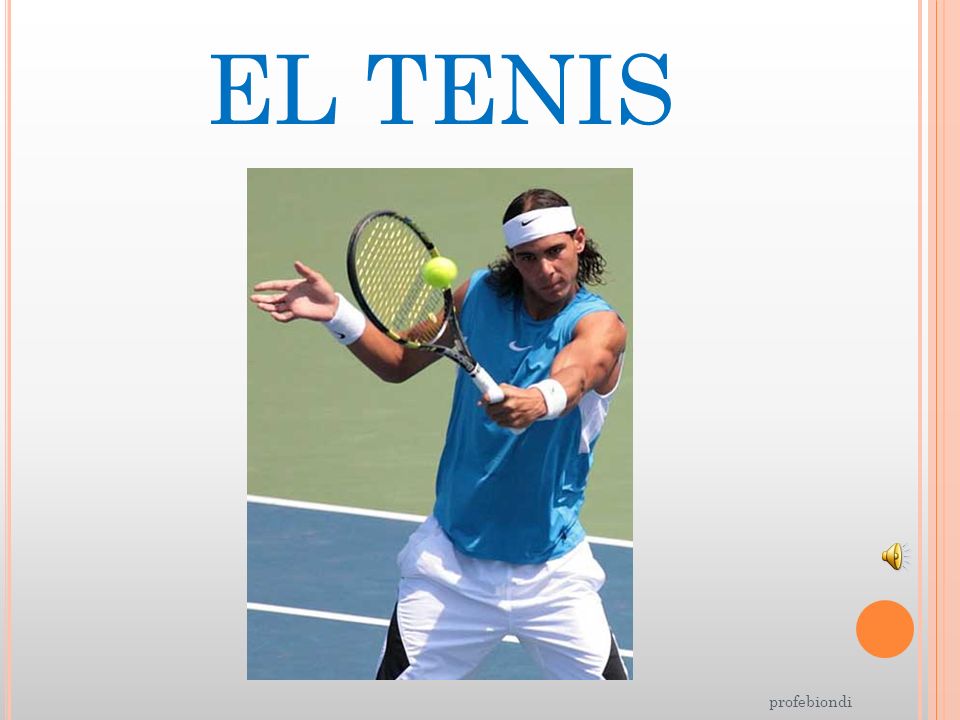The image appears to be a presentation slide, featuring a color photograph centered on a light gray background. The slide is bordered with orange and includes several design elements: a yellow speaker icon at the top left, an orange circle at the bottom right, and the blue text "L TENNIS" prominently displayed above the image. The photograph captures a tennis player in action on a blue and green tennis court with white stripes. The player, wearing a blue sleeveless Nike shirt with a visible white swoosh logo, white shorts with a black design, white Nike headband, and matching white wristbands, has shoulder-length brown hair curling at the ends. He lifts his muscular left arm, poised to strike a bright green tennis ball with his black racket that features yellow accents and a white handle. His right arm is bent and extended to the side. The composition of the slide and the athletic posture of the player create a dynamic and engaging visual representation.